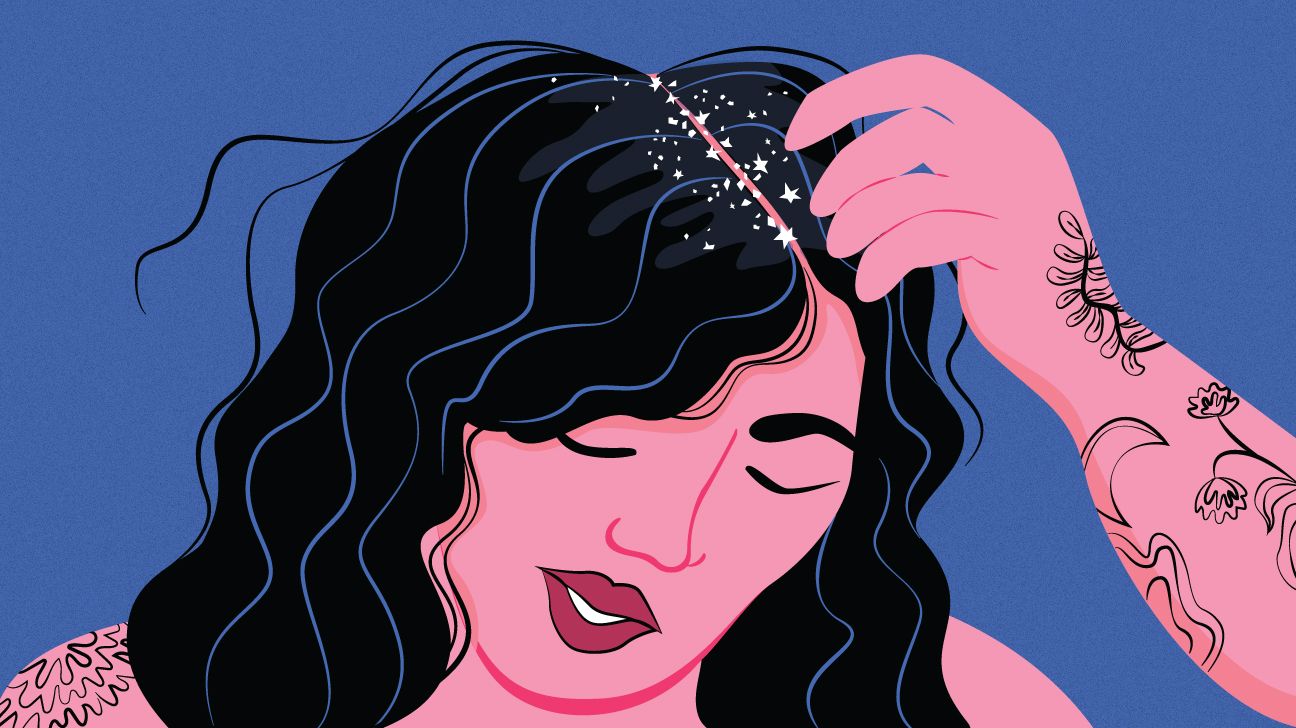This is an illustrated depiction resembling a cartoon version of a woman with distinct and vibrant features. The character has pink skin with a darker pink line representing her nose. Her eyes are closed, depicted by solid black lines for her eyelids, and only one black-painted eyebrow is visible on the right side. The woman's lips are dark purple, outlined in black, and her mouth is slightly open, revealing white teeth. Below her chin, a light pink color differentiates her chin from her chest.

She has long, wavy black hair parted in the middle, with striking blue streaks along the length. A pink line runs along the central part of her hair, which gives her a dramatic appearance. Emerging from the middle part of her hair are small white stars, resembling sparkling starbursts. Positioned to the right, an arm is visible with its pink fingers pointing straight down at the woman's head. This arm, adorned with black plant-like tattoos, including a floral branch, adds to the intricacy of the character's design. The left shoulder, also pink, is decorated with black swirling tattoos.

The entire scene is set against a deep blue background, which makes the vibrant colors of the character stand out even more.